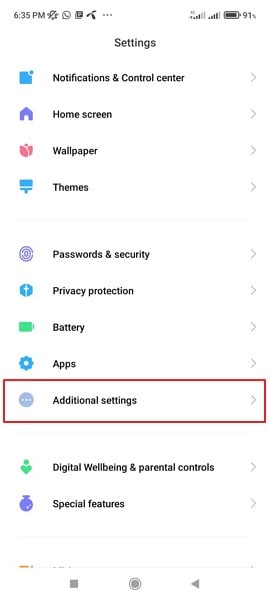The image depicts a phone's settings screen displayed at 6:35 PM. In the top status bar, various indicators are visible: 

- On the right, there are icons for Do Not Disturb, WhatsApp, a square symbol, three leaves, and a three-dot menu. 
- On the left, there is a Wi-Fi icon with signal bars, a network signal icon with four bars, and a battery icon showing 91%.

Below the status bar, the settings menu is listed in the following order:
- Notifications
- Control Center
- Home Screen
- Wallpaper
- Themes
- Password and Security
- Battery
- Apps
- Additional Settings (highlighted with an unnatural red border)

Following this menu, more options are available:
- Digital Wellbeing
- Special settings

The image emphasizes the "Additional Settings" option by enclosing it in a red border, suggesting it has been manually highlighted for emphasis.